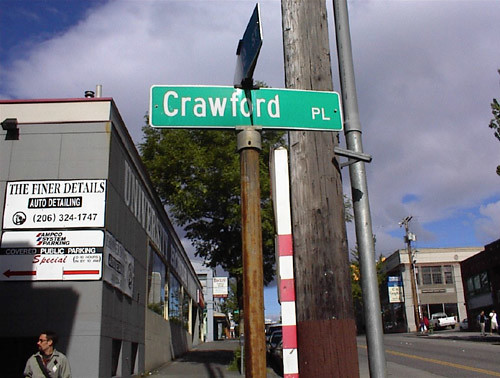The image captures a street corner featuring a prominently rusted, large pole with a green street sign that reads "Crawford Place." The pole intersects with another sign, partially obscured from view. Adjacent to the pole is an aged, dry wooden telephone pole, standing next to a silver pole. On the corner, a gray-colored storefront displays signage for "The Finer Details Auto Detailing" along with a contact number, though it is unclear if the number is part of the building's advertisement. Additionally, the building features the words "University something" in white letters on its facade. A man in a gray shirt and glasses, with an item slung over his shoulder, is walking across the street. The scene also includes various buildings in the background under a gray, overcast sky.